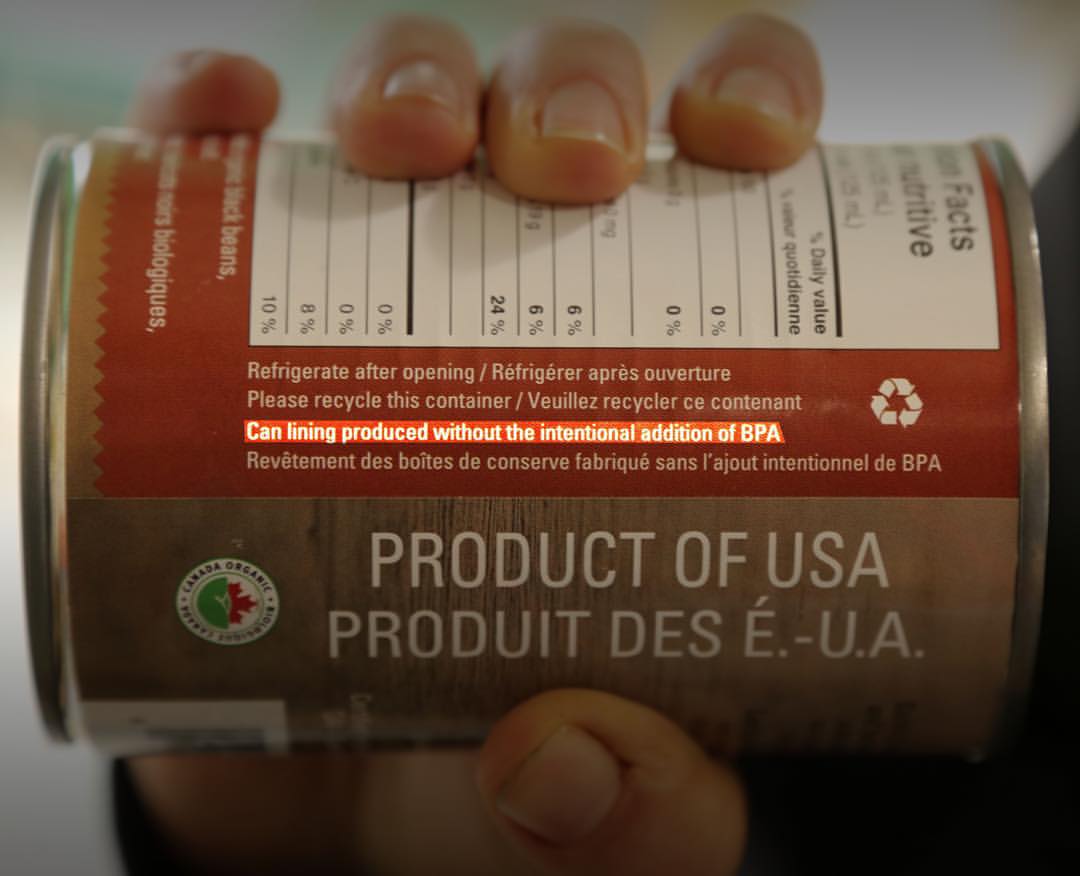A hand, with the thumb supporting the bottom and four fingers balancing the top, holds a red and brown aluminum can sideways, revealing its intricate label details. The can prominently features white text, including a large “Product of USA” label, paralleled by its French translation “Produit des E.-U.A.” Beneath this, a highlighted red section declares, "Can lining produced without the intentional addition of BPA." This is accompanied by a note urging to "please recycle this container" and to "refrigerate after opening." Additionally, a white nutrition facts label is visible amid this bilingual and conscientious design. A logo is visible to the left of the text.